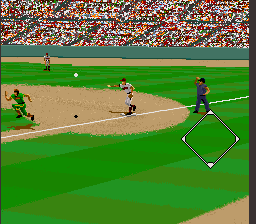The image is a detailed screenshot from a baseball video game. It captures the intense moment of a player sprinting from one base to another, with a catcher from the opposing team positioned to either catch or throw the ball. The player's swift movement and the catcher's poised stance create a sense of high anticipation. In the background, a crowd of spectators is visible, adding to the overall atmosphere even though individual faces cannot be discerned due to the distance. The virtual field and stadium are rendered with impressive detail, enhancing the immersive experience of the game.